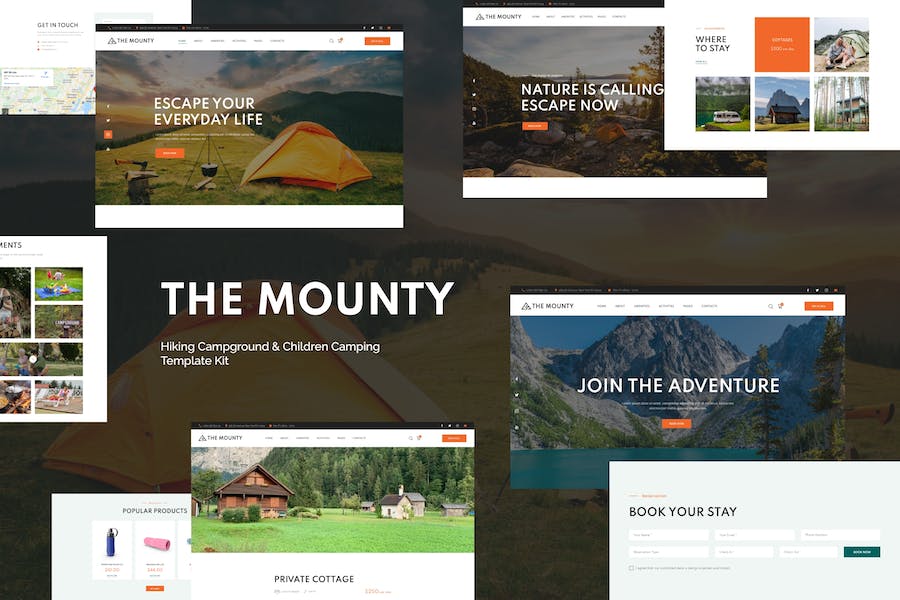This detailed caption describes a screen capture of a camping-themed web page in a landscape orientation, populated with various pop-up windows. The backdrop features a scenic image of a tent set in a picturesque meadow with a backdrop of mountains and trees.

In the top left corner, there's a white pop-up box labeled "Get in Touch." Overlapping this is a larger box that reads "Escape Your Everyday Life," which showcases a tent in a grassy field with mountains and trees in the distant background, framed perfectly to highlight the serene environment.

To the right of this, another box declares "Nature's Calling. Escape Now." It includes an image of what appears to be the same tent set on a rocky surface with a majestic mountainous background, enhancing the adventurous spirit of the content. 

Above this, a third white box is labeled "Where to Stay," featuring a photograph of rustic outdoor buildings, likely intended to provide potential camping destinations.

Below this series of pop-ups, a headline in white text declares "The Mountie," describing it as a "Hiking Campground and Children Camping Template Kit." This part of the page seems to function as an advertisement for a specific camping area or an organized camping template kit.

On the far right, a captivating call to action reads "Join the Adventure," accompanied by an enchanting image of a lake with mountains in the background, creating a sense of allure and excitement for potential campers.

Beneath this, the web page offers an area titled "Book Your Stay," where users can enter search criteria to customize their camping experience, followed by a call-to-action button labeled "Book Now."

Overall, this screen capture effectively conveys a blend of adventure, natural beauty, and practical information, enticing viewers to explore and book their next camping trip.